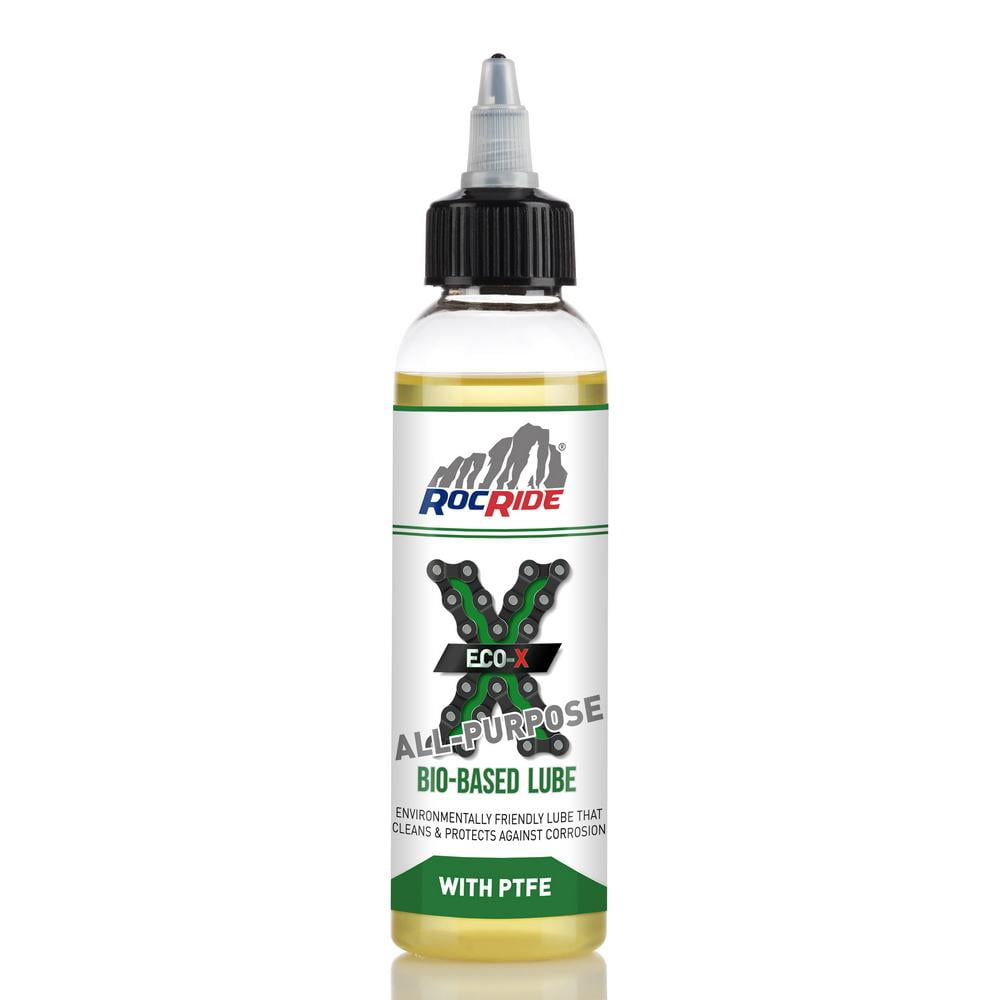This image is a close-up photograph of a bottle of bio-based lubricant, set against a completely white background. The clear, long, and tall bottle is filled with a goldish-yellow fluid. It has a black twist-on cap with a ribbed, white pointy tip, and you can see the black plastic interior of the cap. The label on the bottle prominently features a gray mountain range at the top, under which the brand name "ROC RIDE" is displayed in blue and red letters. Beneath this, there is a green stripe and a large green 'X,' bordered by what appears to be a black and gray bicycle chain. The center of the 'X' is also green, with "ECO-X" written in white and red lettering. Additional descriptions on the label include "ALL PURPOSE" in grey letters, "BIO-BASED LUBE" in green letters, and "ENVIRONMENTALLY FRIENDLY LUBE THAT CLEANS AND PROTECTS AGAINST CORROSION" in black letters. At the bottom of the label, on a green background with white letters, it reads "WITH PTFE."